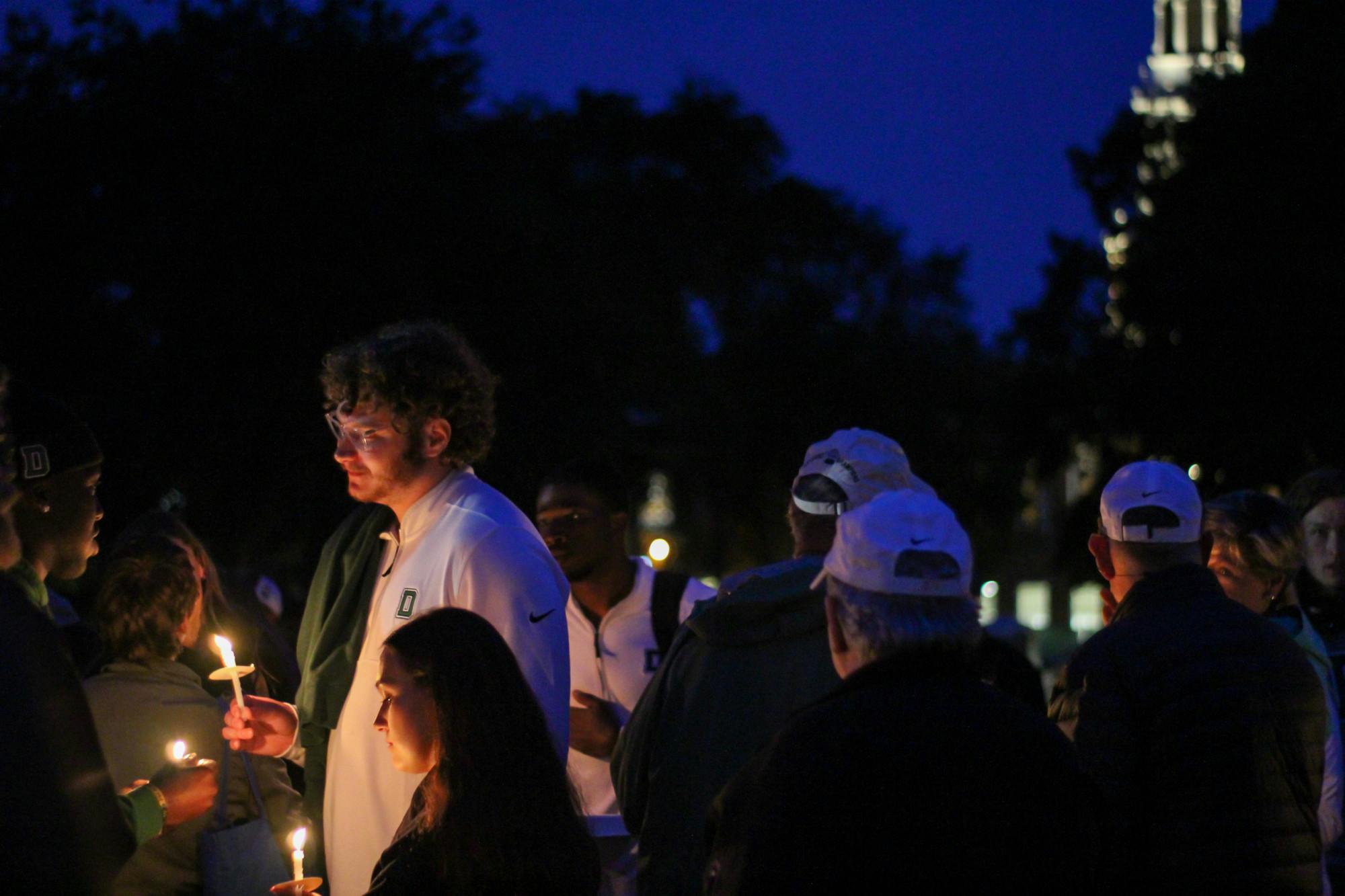This nighttime photograph captures a somber candlelight vigil, held against the backdrop of an illuminated building that resembles a capitol structure. The scene is enveloped by a dark blue sky and silhouetted trees. A diverse crowd of about ten people participates in the memorial, each holding a candle equipped with a wax catcher. The mood is somber as they face various directions, some engaging quietly with each other. Notably, a tall white man with curly hair, a beard, and glasses stands out on the left side, his face solemnly lit by candlelight as he converses with a black man wearing a hat with the letter 'D'. To the right, three men in white Nike baseball caps are also visible among the group. The atmosphere is reflective and respectful, with the candle flames casting a gentle glow on the participants' faces.